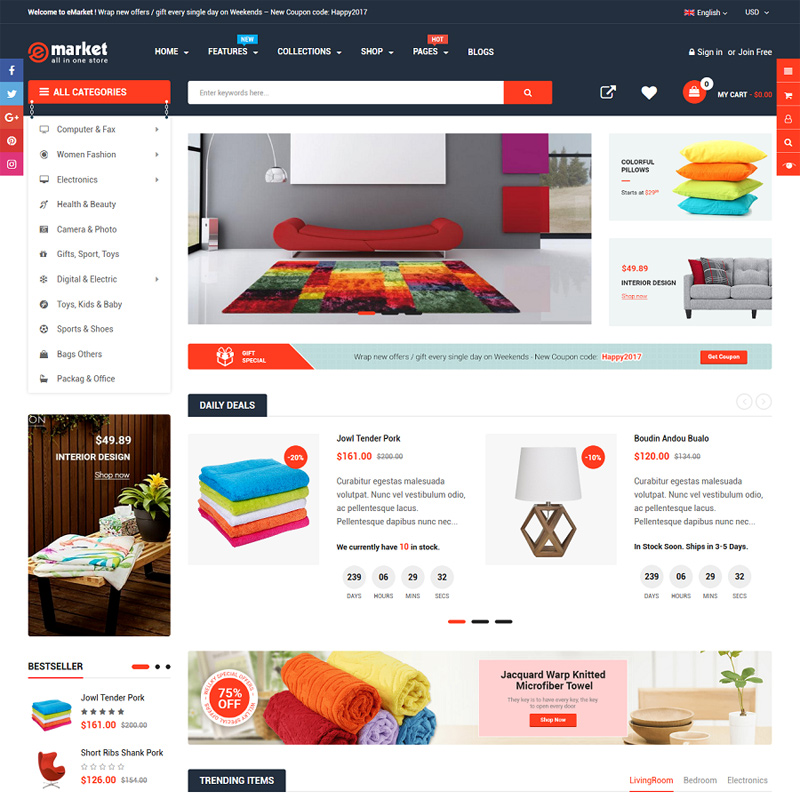The image is a screen capture of a shopping website's homepage. At the top, there is a black horizontal frame featuring the site’s name, "eMarket - All in One Store." The 'E' in "eMarket" is distinctively styled in red and enclosed within a red circle. To the right of the site's name, there is a navigation menu with white text displaying the links: Home, Features, Collections, Shop, Pages, and Blogs. Directly beneath this header is a prominent white search bar.

The main body of the webpage showcases various colorful photographs. Dominating the center is an image of a modern and elegant living room. The space features a shiny white floor and a gray wall, complemented by a striking red contemporary couch. The couch sits on a vibrant, multi-colored, square-patterned rug. To the right of the couch, four colorful pillows are stacked neatly on top of one another, ordered from top to bottom in yellow, orange, green, and blue.